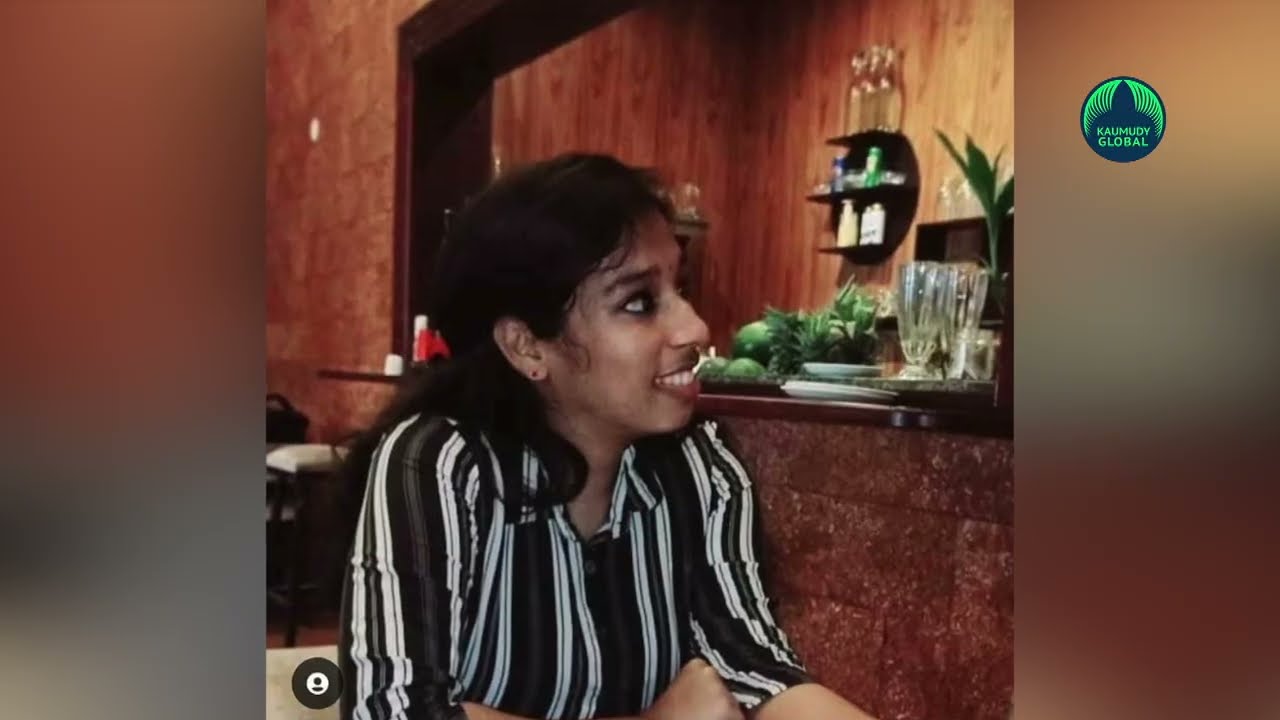The image depicts a young woman, possibly of Indian descent, with medium to dark skin and long black hair that extends past her shoulders, with some strands falling over her shoulder. Her hair appears slightly frizzy and might be tied back into a ponytail. She is seated, likely at a table in a restaurant or cafe. She is dressed in a black and white vertically striped blouse that covers her shoulders and has sleeves rolled up to her elbows, revealing her bare forearms. Around her neck is a gold necklace. The woman is smiling and looking up and to the left, captured in a semi-profile view.

The setting appears to be a restaurant or cafe with a mix of dark stone and brown wooden walls. In the background, there is a bar area displaying trays with various drinks, glasses, and a variety of fruits or vegetables, suggesting it might be a juice bar. The walls behind her have some red and orange tile or marble details. Notably, there is a logo in the top right corner of the image that reads "Kuambai Global," spelled K-A-U-M-U-D-Y, accompanied by a blue pointed spiky object. There is also an insignia visible in the bottom left corner. In the far background, there is a table set for two, adding to the restaurant ambiance.